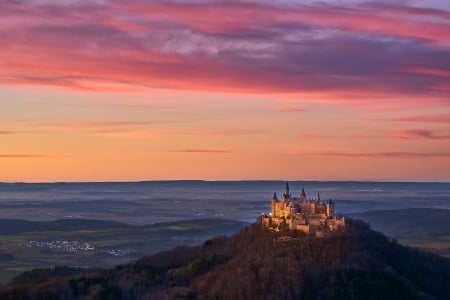This photograph, which could also be mistaken for a painting due to its artistic quality, captures a majestic castle perched atop a rugged hill that overlooks a vast ocean. The castle, bathed in a soft, yellowish-tan light likely enhanced by the setting sun, dominates the rocky mound in the foreground. The terrain around the castle is brown and gray, giving it a stoic, timeless appearance. Clustered houses can be seen dotting a large green expanse between the hill and the ocean shore.

The ocean stretches out toward the horizon, reflecting the rich colors of the sunset. The sky is a dazzling palette of peach, orange, and yellow hues near the horizon, seamlessly blending into dusky gray, pink, and purplish clouds higher up. The cloud line running across the top of the image glows with a reddish tint on the underside, adding to the dramatic ambiance. This stunning scene is framed by the contrasting vividness of sunset colors and the serene blues of the ocean waves, creating a visually captivating and detailed landscape.